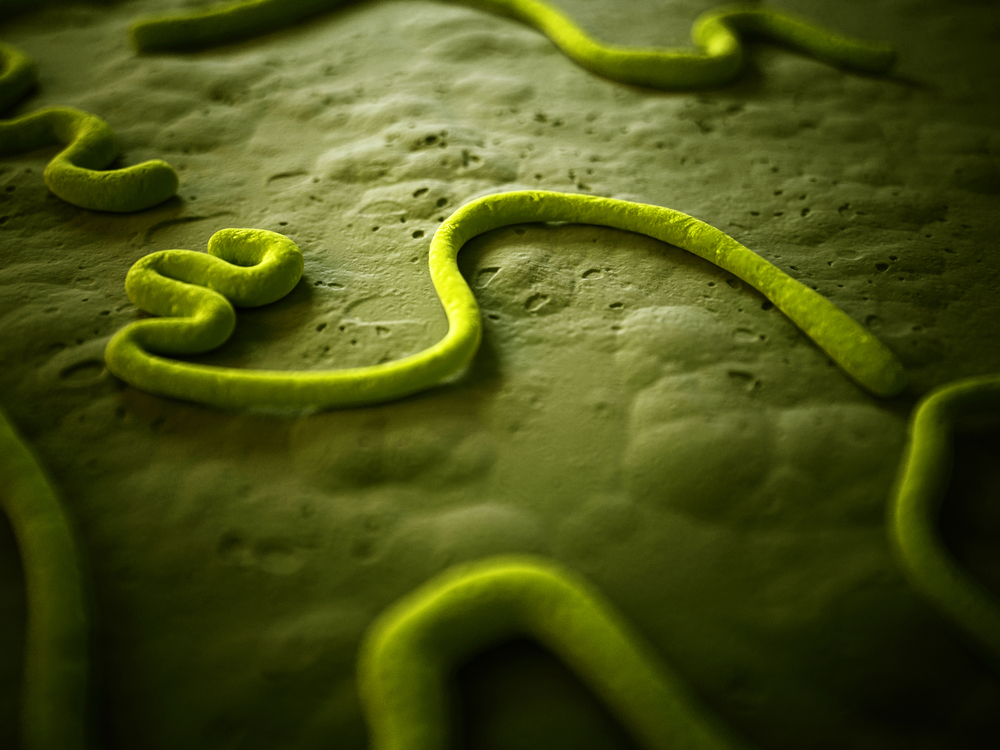The image is a close-up photograph of a roughly textured, dark green surface, reminiscent of a moon-like landscape characterized by small holes, craters, and bumpy protrusions. Scattered across this surface are several worm-like forms, predominantly light green with patches of darker and yellowish green. The forms, resembling Play-Doh or a dough-like material, appear to be curved, with one prominently in focus in the center of the image. This central worm is swirled in a W-like pattern at the top and becomes long and loose towards the bottom. Other similar worms are seen blurred in the background and sides, contributing to an overall scene of various green squiggles on a textured green backdrop.